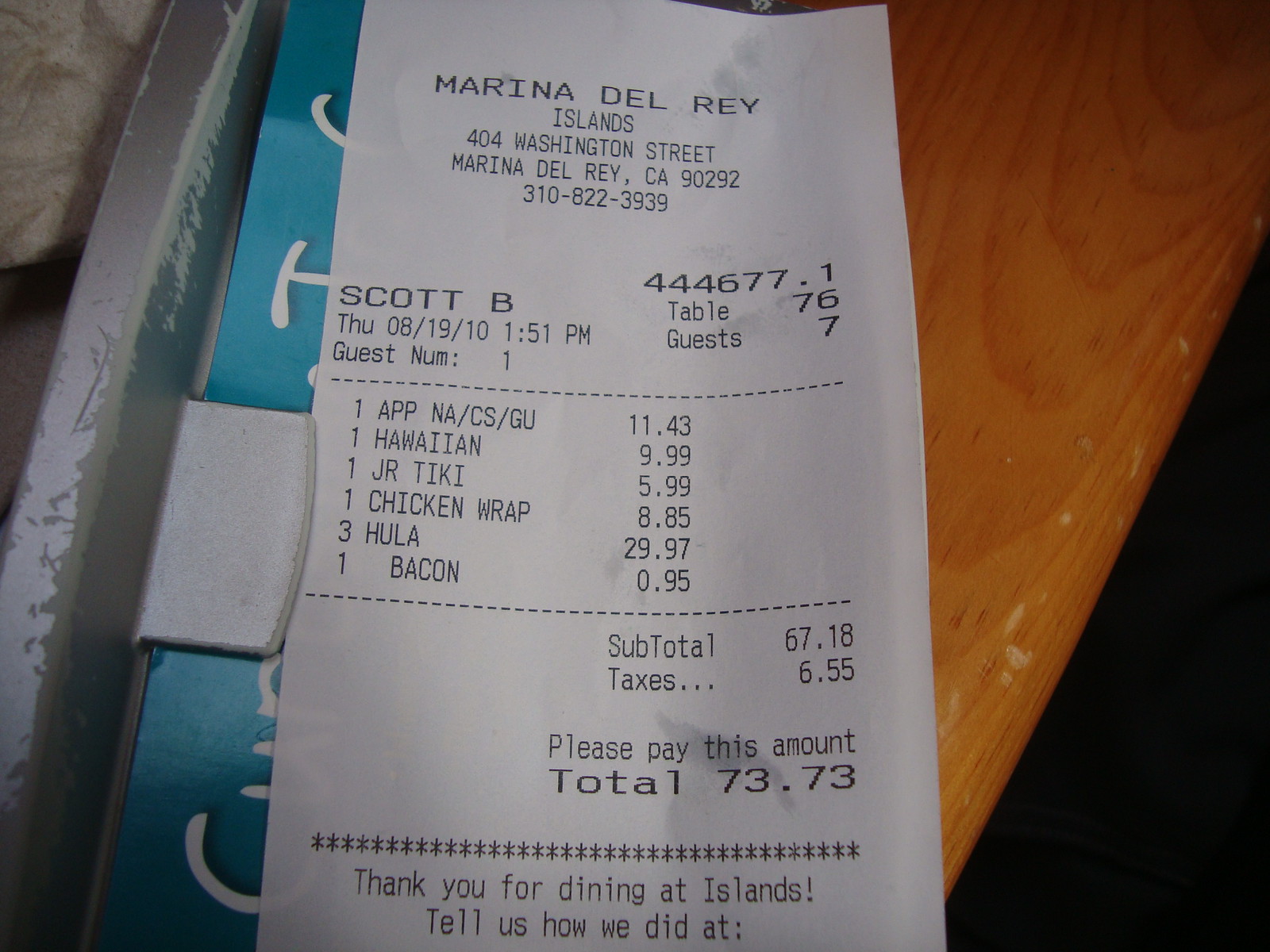This image features a slightly damp receipt from the restaurant Islands, located in Marina del Rey on Washington Street, California. The receipt includes various details such as the zip code and phone number of the restaurant. It lists the order number, table number, number of guests, customer's name, and the date and day of the visit. The items ordered suggest a Hawaiian-style cuisine, culminating in a pre-tax total of $67 and a final amount of $73 after taxes. The receipt concludes with a courteous "Thank you for dining at Islands." The receipt itself is printed on a white background with black text and appears to have been exposed to rain, adding a slightly wet texture to the paper.